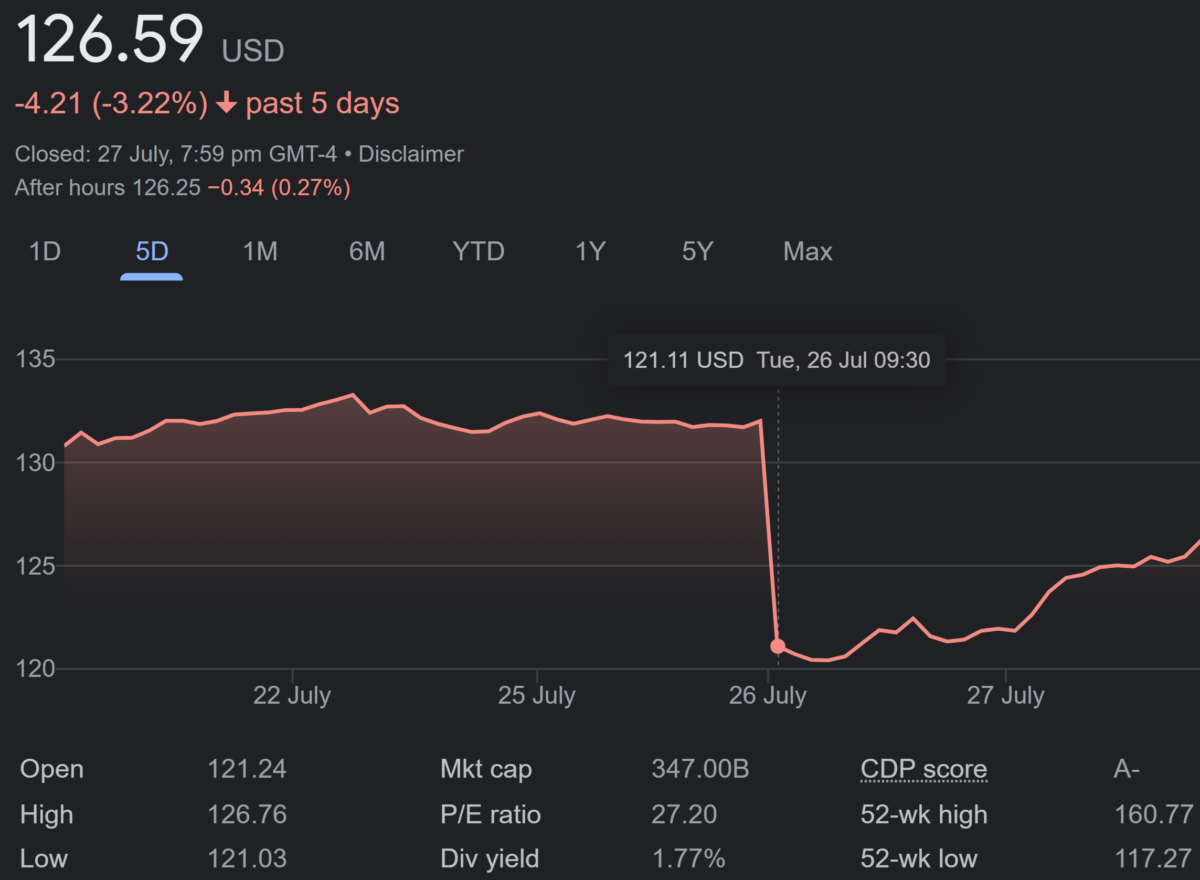A detailed summary of a financial stock image displays key information regarding an unspecified stock on the market. The stock's current price is prominently shown in the upper left corner as $226.59 USD. Over the past five days, the stock has experienced a decline of $4.21, equivalent to a 3.22% decrease. This data is dated July 27th at 7:59 PM GMT-4, accompanied by a disclaimer. In after-hours trading, the stock price further lowered to $126.25, representing a decrease of $0.34 or 0.27%, as indicated in parentheses.

The image includes a line graph illustrating the price fluctuations over different days. The graph reveals that the stock opened at a lower price before gradually increasing. Additional fundamental data are displayed at the bottom of the image, including key financial metrics such as the opening price, high price, low price, market capitalization, PE ratio (price-to-earnings ratio), dividend yield, CDP score, and the 52-week high and low values.